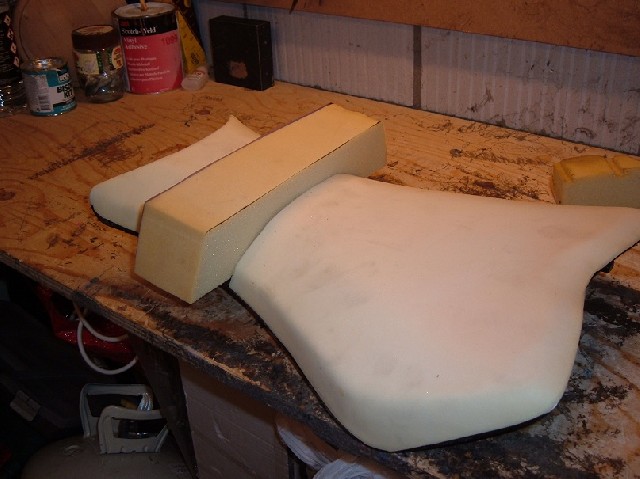The image depicts a cluttered and well-worn workbench, marked with the remnants of numerous projects. The surface of the bench is dotted with a variety of colors, giving it a well-used appearance reminiscent of a chopping block. Dominating the scene, there is a large, bone-white object shaped somewhat like a bicycle seat. On top of this seat-shaped object rests a heavy, gold-colored rectangular block. Surrounding this centerpiece, the background reveals a collection of jars, paint cans, a bottle of glue, and what might be a Wi-Fi box. The workspace is notably messy, with various items strewn both on and under the table, contributing to an overall impression of a busy and industrious area filled with a mix of tools and miscellaneous items.